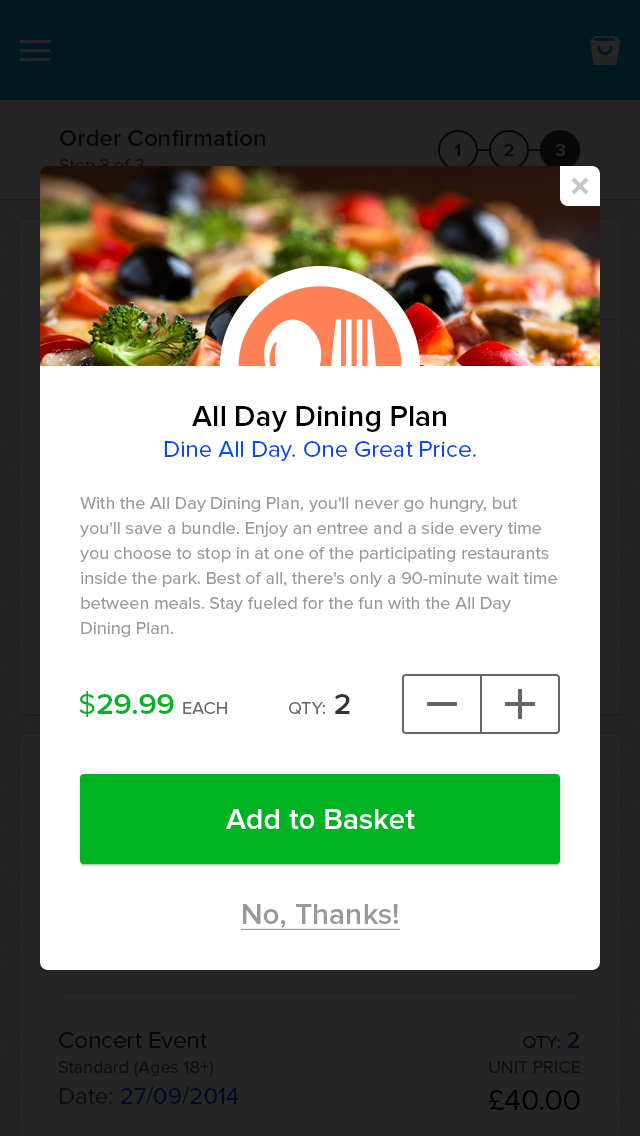Here is a clear and detailed caption for the image:

---

This screenshot appears to be taken from a mobile device, likely a phone or tablet. The background features a top blue bar, with three short horizontal white lines on the far left, possibly indicating a menu icon. To the right, there is an icon resembling a bin or a folder. Below this, in black text, the heading "ORDER CONFIRMATION" is visible. Next to the heading are three numbered circles: '1', '2', and a blackened '3', suggesting the user is at step three of the process.

In the foreground, an overlay window displays an image of a vegetable-topped pizza, accompanied by the text "ALL-DAY DINING PLAN" in black. Beneath this, the phrase "Dine all day, one great price" is highlighted in blue. The description elaborates that the plan allows patrons to enjoy an entrée and a side with every visit to participating restaurants inside a park, emphasizing savings and a 90-minute interval between meals. The plan is priced at $29.99 each, with a quantity of two selected.

Further down, green and grey buttons offer the options "ADD TO BASKET" and "NO THANKS," respectively. At the bottom of the screenshot, there is an indication that the user is booking for a concert event scheduled on 27th September 2014. The event has a quantity of two tickets selected, each priced at 40 euros.

---